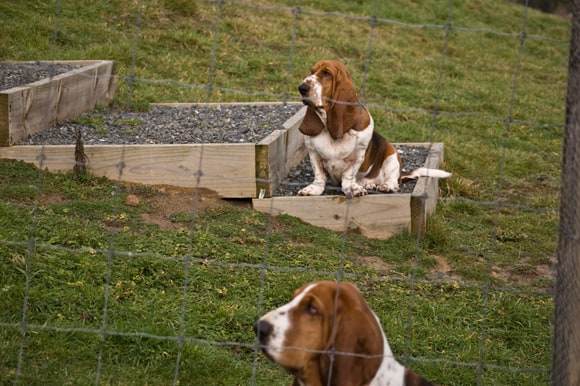In this outdoor daytime image, we see two Basset Hound puppies in what appears to be a backyard or farm setting. The backdrop consists largely of green, albeit somewhat neglected grass, with a glimpse of wooden steps featuring stone and gravel in the upper left corner. The puppies are positioned behind a chicken wire fence, with one puppy fully visible standing on the wooden structure filled with gravel rocks, while the face of the other is visible peeking from behind. Their attention is directed towards something off to the left of the photo. The primary colors evident in the image are shades of green, gray, brown, white, black, and silver. Overall, no text is present, and the image evokes a serene outdoor scene with two attentive puppies as the central focus.